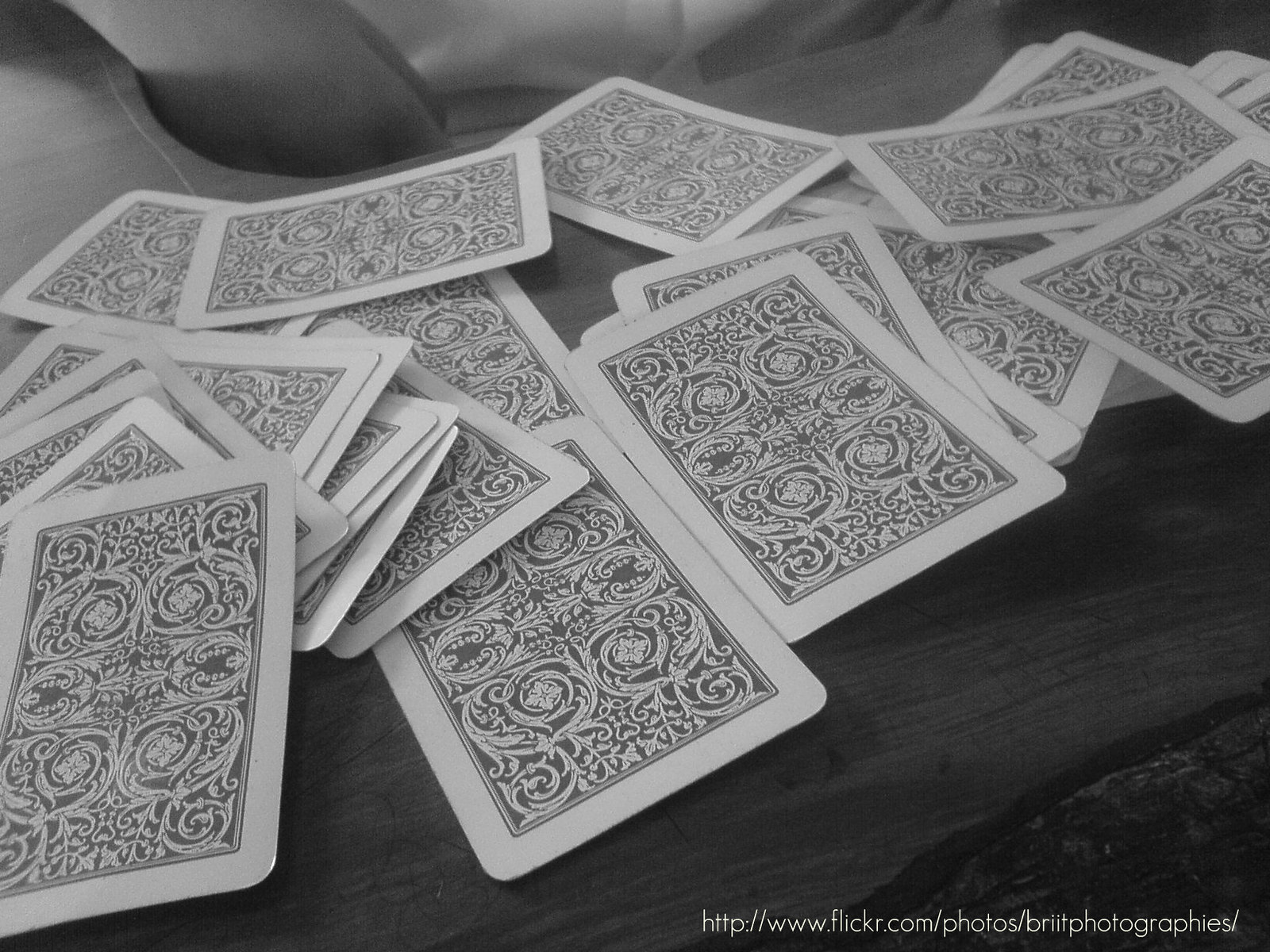A monochromatic photograph captures a disarray of playing cards, all face down, scattered chaotically across a wooden surface. The table, which does not follow a rectangular form, is marked by a prominent crack at the lower right corner, suggesting either damage or its edge. Light and shadow interplay vividly, despite the absence of color, casting varying shades across the scene. Between 20 and 30 cards lay jumbled atop one another without any uniformity, revealing only their backing design. The upper left corner of the table curves, partially obscuring an indiscernible object behind it. In the bottom right corner, a URL indicating the photo's origin is visible: www.flickr.com/photo/photography/...